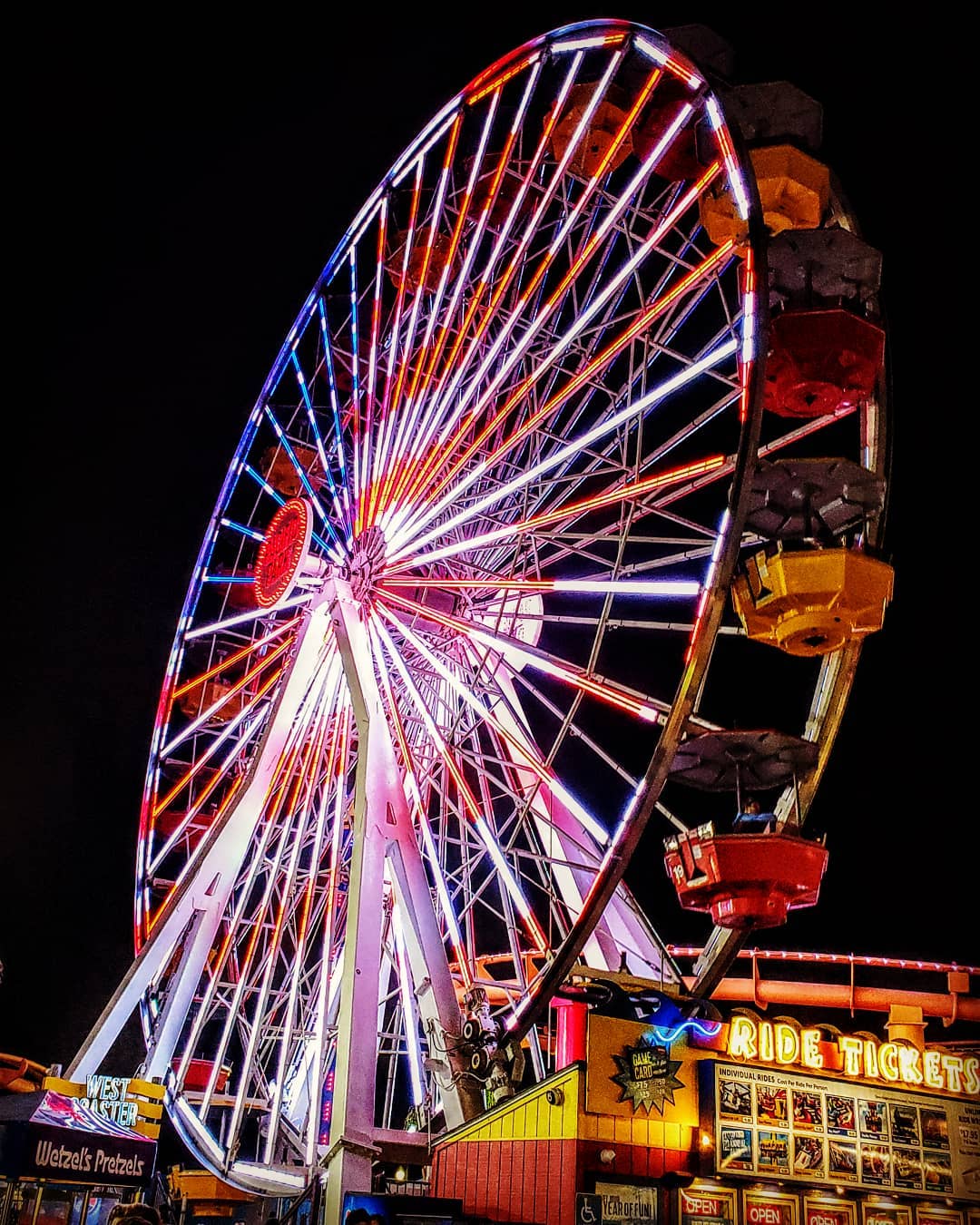This vertically rectangular, full-color photograph captures a vibrant nighttime scene at a carnival, illuminated exclusively by artificial lighting against the backdrop of a solid, black night sky. Dominating most of the frame is a spectacular Ferris wheel adorned with red, white, and blue lights, reminiscent of the American flag. The Ferris wheel's spokes create a dazzling pattern, with cars in various colors including yellow, red, and brown, some of which are occupied by visitors enjoying the ride.

In the lower portion of the image, the ticket booth on the right stands out with its bright, neon "Ride Tickets" sign glowing in yellow light. To the left, partially visible, is a Wetzel's Pretzels stand, adding to the bustling, festive atmosphere typical of a carnival setting. The overall scene suggests a lively, welcoming environment, drawing people into the excitement of the rides and the charm of the food stalls.